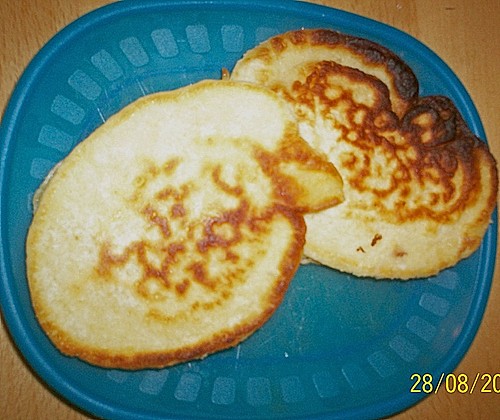This photograph features two irregularly shaped pancakes resting on a blue, square-like plate with rounded corners and decorative edging. The blue plate, which appears to be either plastic or paper, is set against the solid medium brown backdrop of a wooden table. The pancakes, contrasting in their marbled appearance of golden brown with hints of overcooked darker spots, lie with one slightly overlapping the other. The top pancake has a distinct formation that resembles a bird's beak. In the lower right corner of the image, there is a partially cut-off yellow date stamp: 28-8-20. This close-up shot captures the intricate details of the scene, suggesting a casual, homey setting.